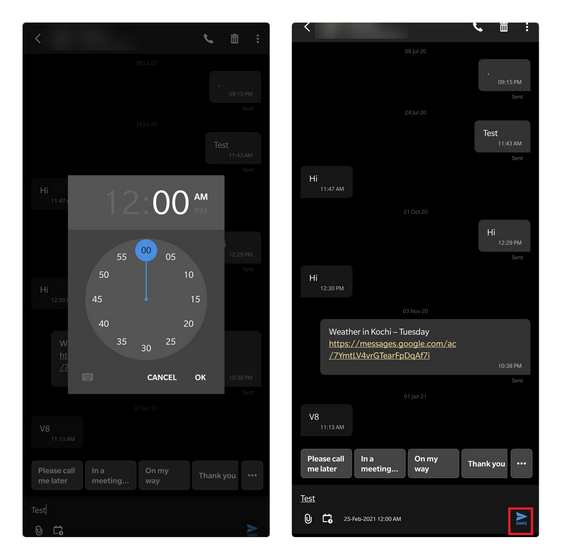Here are two horizontally aligned mobile screenshots, their respective operating systems indeterminate. Both screenshots contain a leftward-pointing arrow, a phone icon, a trash can icon, and a menu represented by three vertical dots. The background of each image shows fragmented conversation bits, mainly repetitions of "test" and "hi," mixed with arbitrary timestamps and seemingly automated messages.

The left screenshot captures a clock interface set at 12 a.m., though it allows switching to p.m. Users can adjust the time by dragging their finger around the clock face, which displays numerals in increments of five minutes from 5 to 55. Alternatively, a keyboard can be summoned for direct time entry. Below this interface, quick message options are visible, including "Please call me," "Later," "In a meeting," "On my way," and "Thank you." A test message can be seen typed out near a microphone, a calendar icon, and a send button.

The right screenshot focuses more on a conversation timeline. It details specific exchanges: a "test" message at 11:43 a.m., followed by a "hi" at 11:47 a.m., continued by repetitive greetings ("hi") exchanged on October 21st, 12:29 p.m., and 12:30 p.m. A message referencing the weather and a garbled Google Messages URL appears on November 3rd, 2020 at 10:38 p.m. Further testing is indicated to occur on February 25th, 2021 at 12 a.m. The sequence suggests an ongoing evaluation of a chat app potentially featuring scheduled messaging.

This detailed breakdown highlights a probable test scenario within a messaging application, demonstrating both manual and automated functionalities with intricate timestamps and varied preset message options.